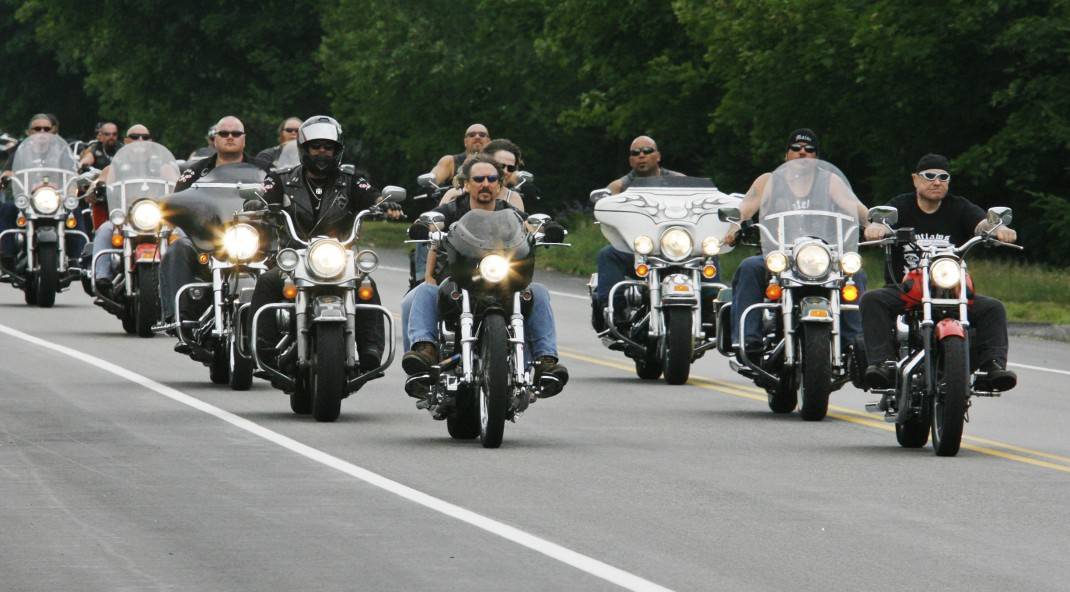In this outdoor daylight image, a group of about 12 to 15 bikers are riding their Harley Davidsons down a two-lane highway. The scene captures a diverse array of motorcycles, each with distinct handlebars—some wide, some narrow—many equipped with windshields and all with their headlights turned on. The bikers themselves present a varied appearance: some wear helmets, others opt for hats or bandanas, and most don sunglasses. They are uniformly dressed in jeans of varying colors, complemented by assorted shirts and predominantly black leather jackets. The highway is marked by a central yellow line and flanked by two white lines, which run parallel on either side of the road. The surrounding environment is lush with greenery; trees and grass populate the scene behind the motorcyclists and to the right side of the road, suggesting a rich, natural backdrop. Despite the daylight, the sun does not seem to be shining, giving the image a somewhat muted lighting.